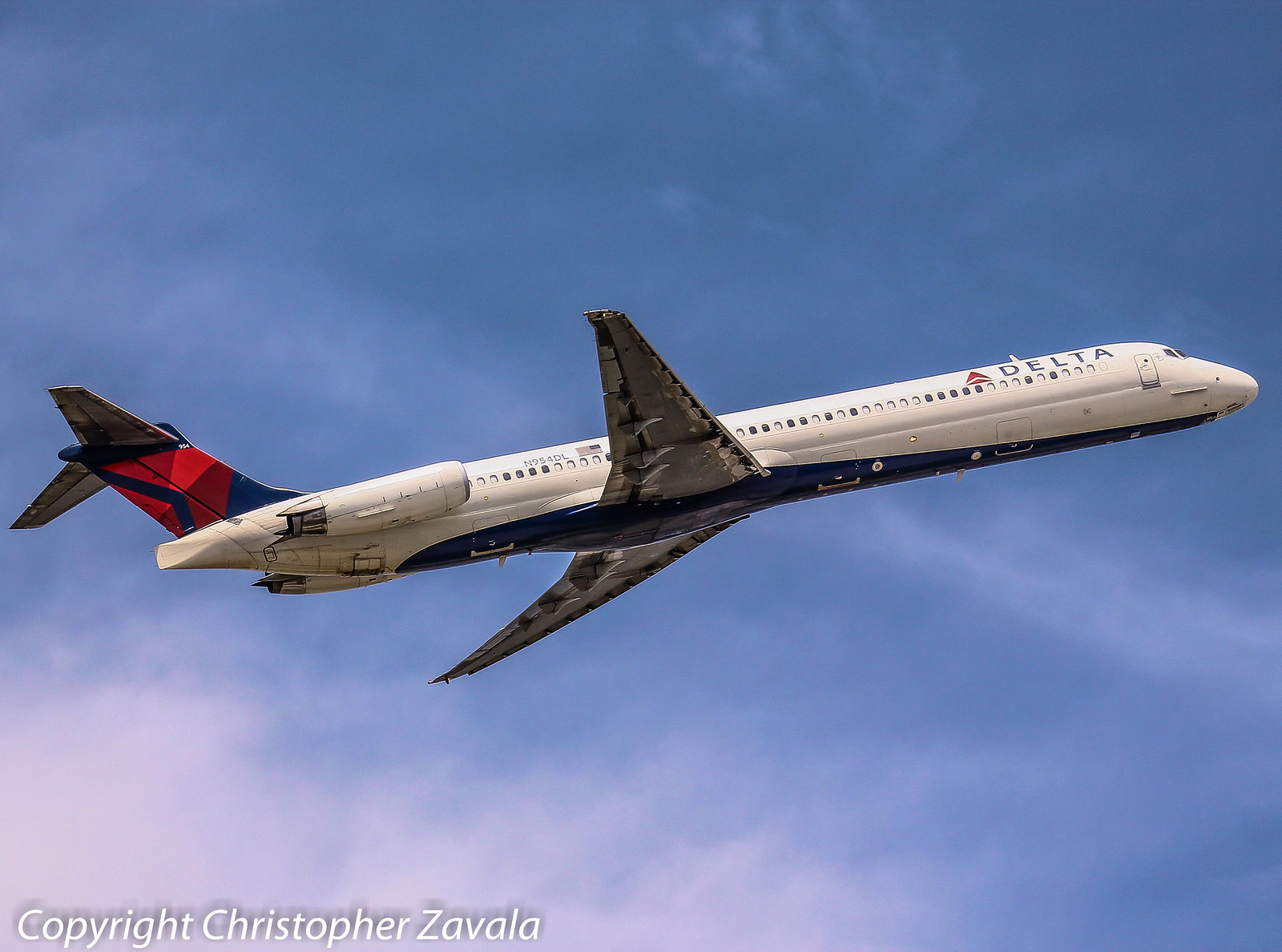This professional photograph by Christopher Zavala captures a Delta commercial airplane in flight, shortly after takeoff. The plane is predominantly white with a distinctive Delta logo on its tail, which is colored red and blue. Beneath its wings, which are a metallic gray, there are two rear-mounted engines. The sky behind the airplane is a mix of crystal blue with wispy white clouds, while more substantial puffy clouds are visible in the lower left corner, near the copyright notation. The aircraft appears relatively large, suggesting it could accommodate up to 300 passengers. Notably visible are the front exit door near the cockpit and two windows in the cockpit itself. The captivating image, which may serve well for advertising purposes, evokes a sense of grandeur and engineering marvel in modern aviation.